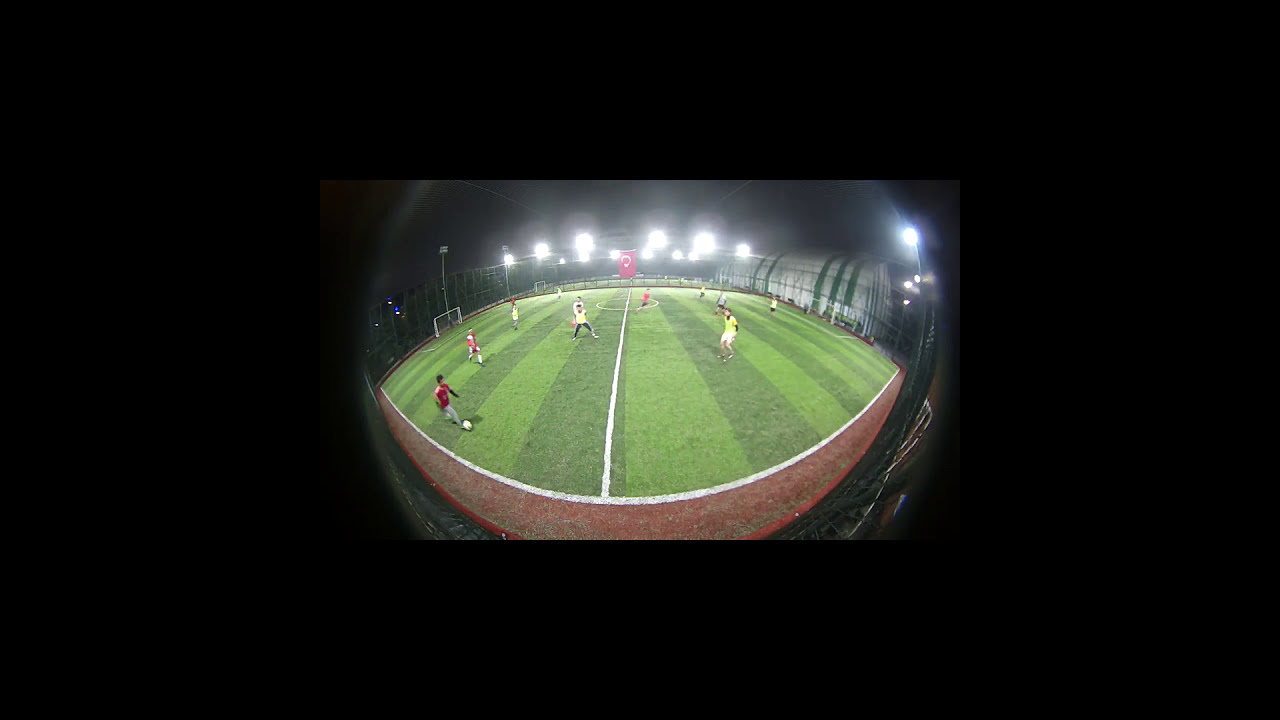This image, captured through a fisheye lens, depicts a dynamic soccer match taking place on a brightly lit grass field under a night sky. Despite the slight distortion from the fisheye effect, the scene is clear: two teams are in the midst of an intense game, with players donning red and yellow uniforms. A player in a red jersey is prominently seen controlling the white soccer ball, directing it upwards across the field. The presence of a referee indicates that this is a competitive and official match, although the exact score remains unknown as there is no visible scoreboard. In the background, a significant structure looms, likely part of a large sports complex, complete with a fence enclosing the field. A red flag emblazoned with a "C" and a star is prominently displayed in the center of the image, possibly indicative of a country or team symbol. Additional fields and a large white and green object are visible in the distance, further emphasizing the size and scope of the sports facility. Spectators, if present, are not discernable due to the distance, but the focus remains on the players eagerly anticipating the next move in this well-lit, night-time soccer game.